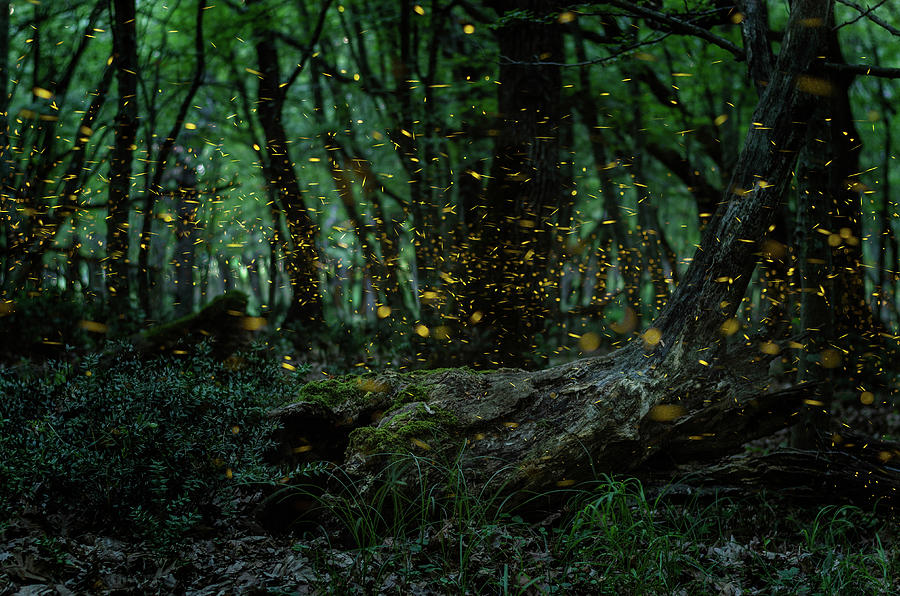An enchanting and somewhat mystical scene depicts a dense forest teeming with thick and thin tree trunks stretching upwards, their dark forms contrasting against a predominantly green background suggestive of lush foliage. The foreground features a fallen tree trunk lying across the ground, surrounded by abundant greenery. The image, an intricate stylized illustration rather than a real photograph, has an air of mystery heightened by the twilight setting. Scattered throughout are numerous gold specks, resembling flickering fireflies, adding a magical touch. These tiny specks vary in form, including circles akin to gold coins, lines, and dots. The forest, shrouded in darkness and devoid of visible inhabitants, hints at the possibility of an AI-generated creation, blending reality and fantasy in a captivating manner.